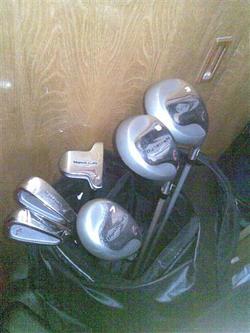The image depicts a slightly downward perspective of a black golf bag containing a mix of six golf clubs, each with visible metal heads. The bag appears to be glossy black and features a strap handle over the top. Among the clubs, three have broad, round, silver heads with black markings, while two have smaller, pear or teardrop-shaped heads with silver and white markings. There is another club with a short crossbar. The golf bag is standing upright, leaning against or in front of a blonde wooden cabinet door, which has a visible handle on the upper right side. Details of the wood grain are noticeable, suggesting the cabinet could be some sort of locker. The lower part of the image is slightly blurred, showing a gray surface that could be either concrete or carpet. No additional background details are clear.